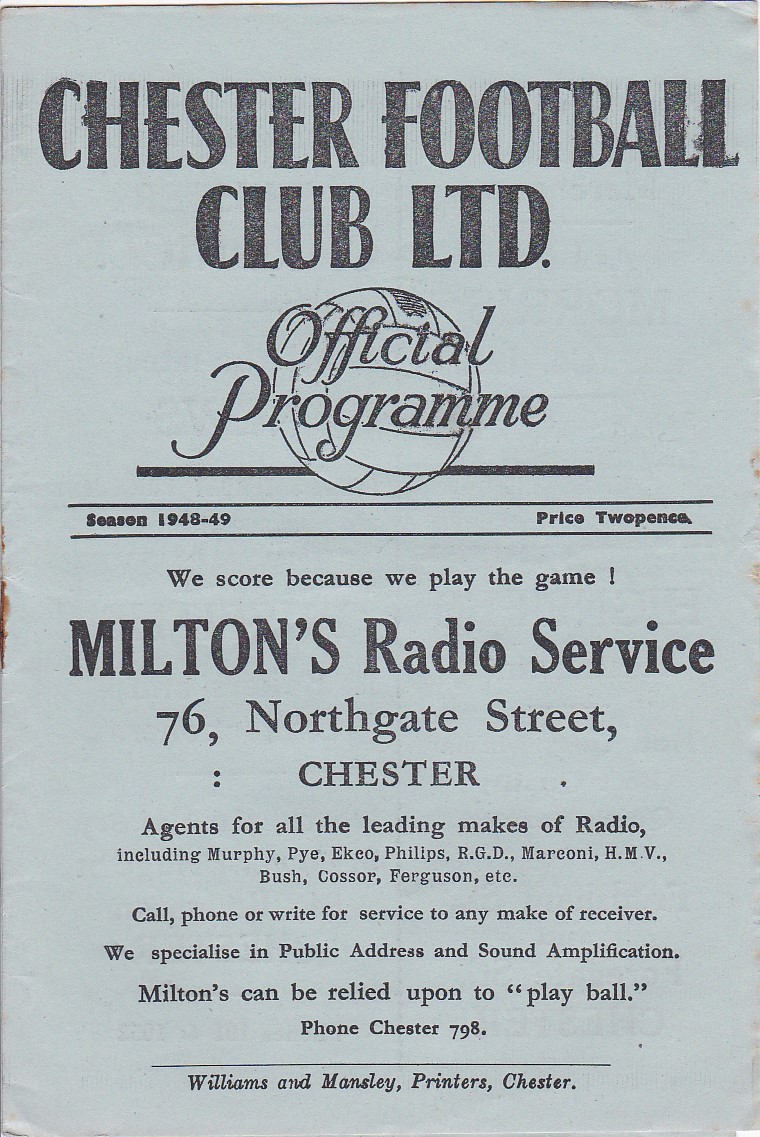This image depicts the front cover of a vintage Chester Football Club LTD official program for the 1948-49 season. The well-aged program, priced at two pence, features a prominent black and white layout with large bold text at the top declaring "Chester Football Club Limited." Below, set within an image resembling a volleyball, the words "Official Program" are inscribed, followed by two lines denoting the season (1948-49) and the price.

The central motto, "We score because we play the game," leads into an extensive advertisement for Milton's Radio Service, located at 76 Northgate Street, Chester. Milton's advertises itself as agents for all leading radio brands including Murphy, Pi, Echo, Phillips, RGD, Marconi, HMV, Bush, Kosser, and Ferguson, among others. The text encourages potential customers to call, write, or phone for service for any make of receiver, noting their specialization in public address and sound amplification. They assert their reliability with the statement, "Miltons can be relied on to play ball," and provide a contact number, Chester 798.

The cover shows signs of its age, with rust stains from staples visible on the left and center, and additional marks on the right suggesting water damage and general aging. The overall color is described as predominantly blue with tones of gray, indicating a well-preserved yet antiquated piece of memorabilia. The program was printed by Williams & Mansley's Printers in Chester.